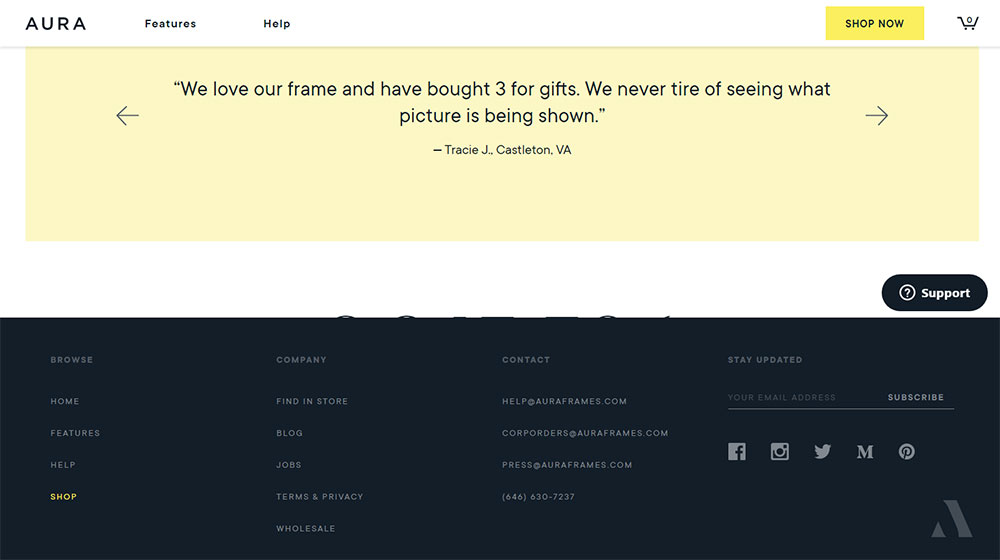A screenshot from the Aura website showcases a variety of navigational and informational elements. At the top of the page, there are navigation links for "Features," "Help," and a prominent yellow "Shop Now" button positioned to the right. Next to it is a shopping cart icon indicating there are zero items in the cart.

Below these elements lies a large, yellow banner with forward and backward arrows on either side, likely used for cycling through different quotes or testimonials. Displayed in the center of the banner is a customer testimonial that reads: "We love our frame and have bought three for gifts. We never tire of seeing what picture is being shown." This quote is attributed to Tracy J. Casselson from Virginia.

In the bottom right corner of the screen, there is a "Support" button with a capsule containing a white question mark. The footer of the page, which is notably tall, contains several columns of links and information. Starting from the left, the columns are labeled:

1. **Browse**: Contains links to "Home," "Features," "Help," and "Shop."
2. **Company**: Includes "Find a Store," "Blog," "Jobs," "Terms," "Privacy," and "Wholesale."
3. **Contact**: Lists an email address, another contact for Corporate, a Press contact, and a phone number.
4. **Stay Updated**: Provides a field to enter your email address and a "Subscribe" button, accompanied by social media icons (Facebook, Instagram, Twitter, an unidentified 'M', and Pinterest).

At the bottom right corner, there is a modern-looking Aura logo, different from the "A" seen in the title bar.

This detailed layout emphasizes the user-friendly and modern design of the Aura website, highlighting its navigational ease and accessibility to customer support and additional company information.